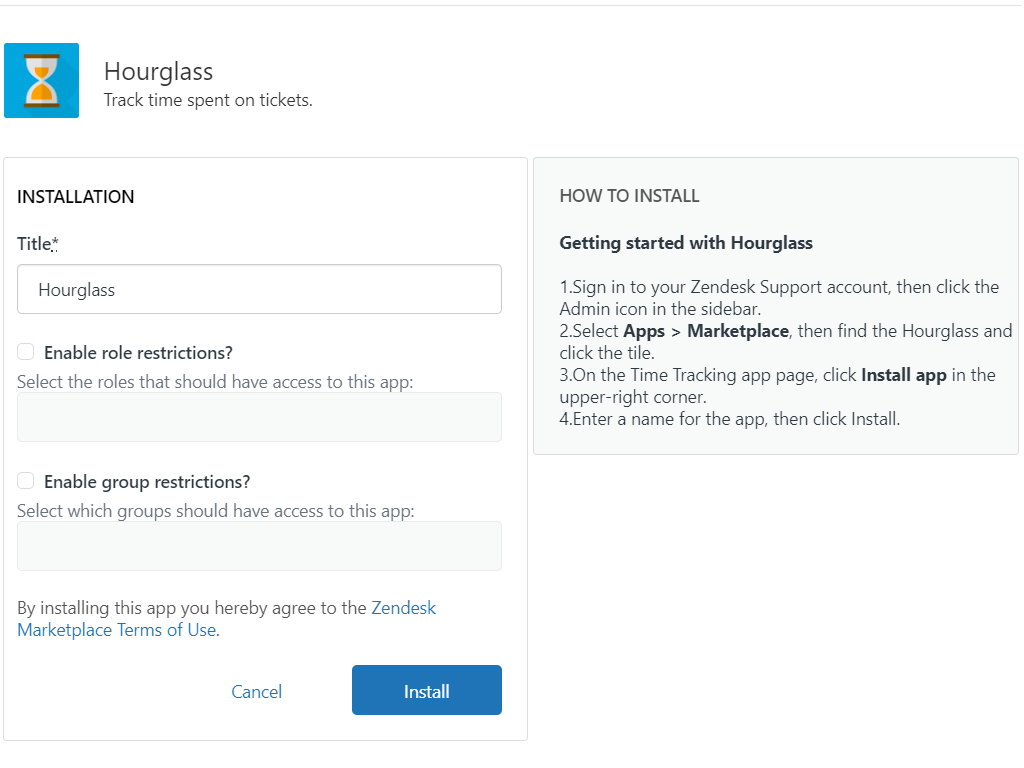This image, taken from a top-down perspective, features a teal-colored box displaying an hourglass filled with orange sand. The sand has accumulated at the bottom, though a portion remains in the upper chamber, ready to trickle down. Below this box, the image is divided into two vertical rectangles: one on the left with a white background and the other on the right with a gray background.

In the white section, there is a title area labeled "Installation," with the word "hourglass" typed in. Below it, a checkbox option reads "Enable role restriction," followed by directions: "Select the roles that should have access to this app." Beneath this, another option, "Enable group restrictions," is presented along with guidance to "Select which groups should have access to this app." Further down, a disclaimer states, "By installing this app you hereby agree to the Zendesk Marketplace terms of use," with a clickable link in blue text enabling the user to read the full terms. At the bottom of this section are clickable options for "Cancel" and "Install," the latter highlighted in blue.

In the gray section to the right, a header reads "Getting Started with Hourglass," and it appears to contain step-by-step instructions for installing the app.